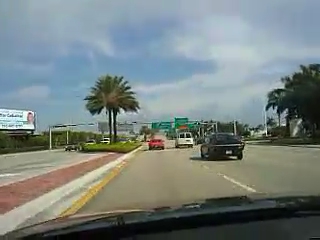This photograph captures a busy street scene from the perspective of a driver seated inside a vehicle. The road appears to be a multi-lane highway, possibly consisting of three lanes in each direction, separated by a grassy median adorned with tall palm trees. Directly ahead of the photographer's vehicle is a red car occupying the same lane. To the right of the red car, in the adjacent lane, there is a black car followed by a white van further up the road. On the far left of the image, beyond the median, a large billboard stands prominently, displaying content in the distance. Additionally, green highway signs are visible further along the road, providing direction to travelers. The sky overhead is a serene blue, dotted with scattered white clouds, adding to the overall vibrancy and liveliness of the scene.